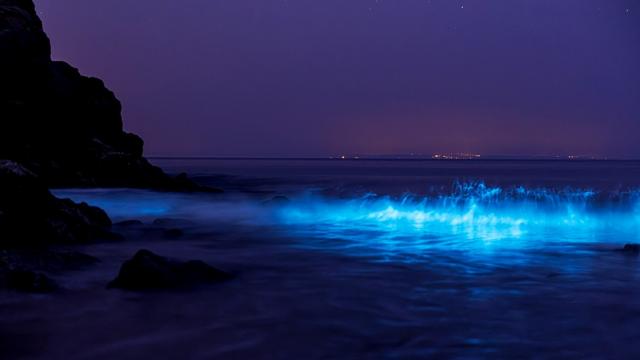This detailed, long exposure photograph captures a mesmerizing nocturnal scene of a rocky shoreline bathed in ethereal light. Central to the image is a glowing, fluorescent blue wave, crashing in from right to left and highlighted by a brighter, almost white core, possibly due to bioluminescent algae. This luminescence accentuates the wave's circular arc, creating a vivid focal point in the middle of the composition. To the left, stark silhouettes of rocky cliffs rise dramatically against the deep purple sky, which transitions into lighter hues of purple and dull red near the horizon. Across the bay, distant lights, possibly of a town, a building, or a bridge, dot the far landmass, adding depth to the scene. The water, otherwise a dark blue, is intricately illuminated by the glowing wave, blending natural beauty with a surreal, almost otherworldly ambiance.